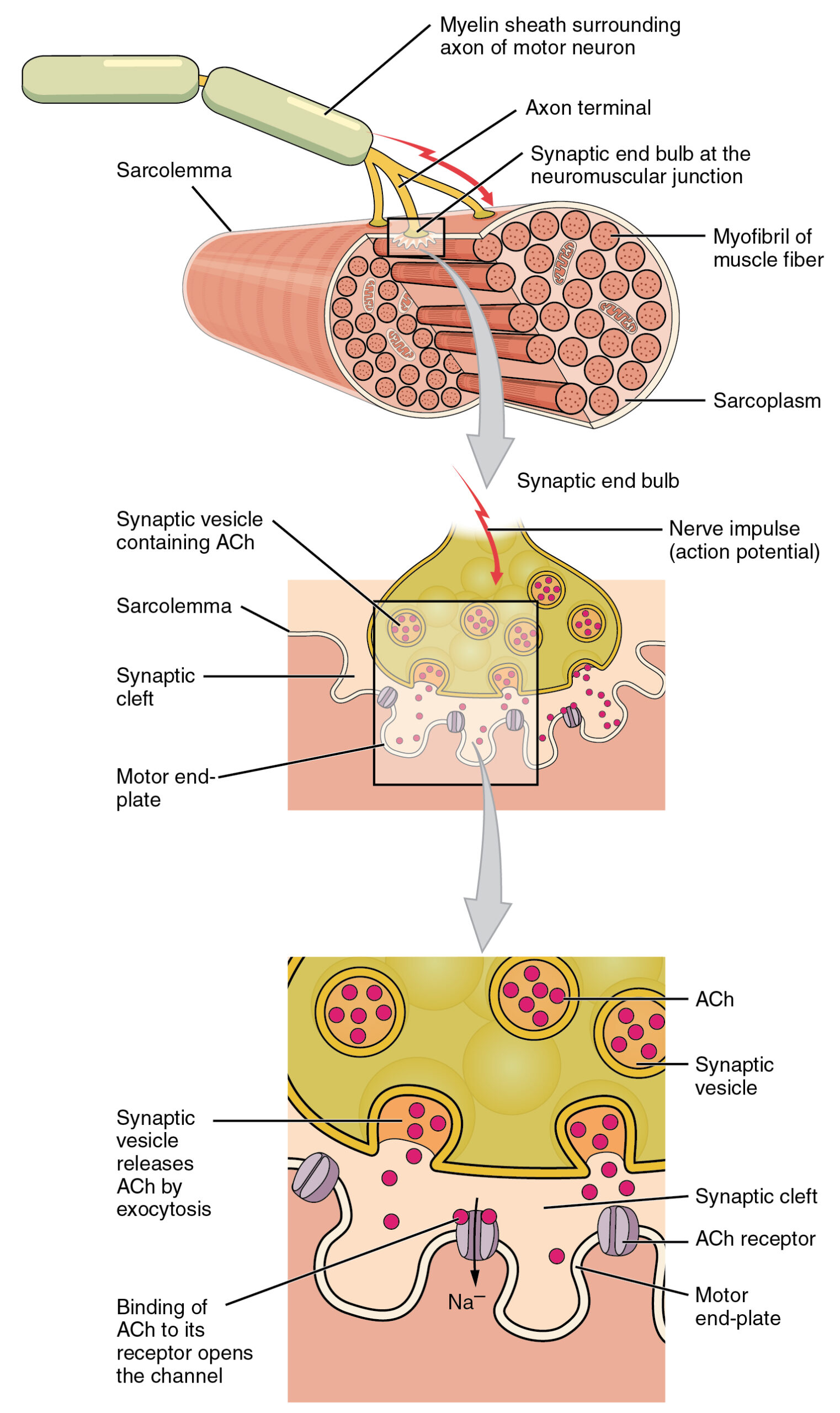The image comprises three distinct diagrams detailing the components and functionality of a motor neuron and its connection to muscle fibers at the neuromuscular junction. 

In the top illustration, a neuron is depicted with several labels pointing to its key parts. The neuron features green myelin sheaths, shaped like elongated capsules, which encase the axon of the motor neuron. Arrows denote different sections: for instance, the sarcolemma is identified at the outer layer, and yellow strands marked as axon terminals culminate in synaptic end bulbs at the neuromuscular junction. These synaptic end bulbs, containing red, dotted synaptic vesicles within an orange oval structure, release acetylcholine (ACH) and interface with the red muscle fiber. Surrounding the myofibrils within the muscle fiber, the substance is termed sarcoplasm. Key anatomical labels include the synaptic cleft, motor end plate, and nerve impulse action potential.

The middle diagram zooms in on a section emphasized in the top image, focusing on the synaptic end bulb's interaction with the muscle fiber. Detailed labels indicate the presence of synaptic vesicles containing ACH, the sarcolemma, and the synaptic cleft. The motor end plate and nerve impulse action potential mechanisms are also highlighted.

The bottom diagram provides an even closer look at the synaptic end bulb region, specifying the process of ACH release by exocytosis. This image emphasizes the binding of ACH to its receptor, opening the channel for neurotransmission. The synaptic cleft is depicted as a pink area, while gray circles with a central line illustrate the ACH receptors, underlining the crucial interface at the motor end plate.

Together, these illustrations intricately convey the neural mechanisms facilitating muscle contraction at the cellular level.